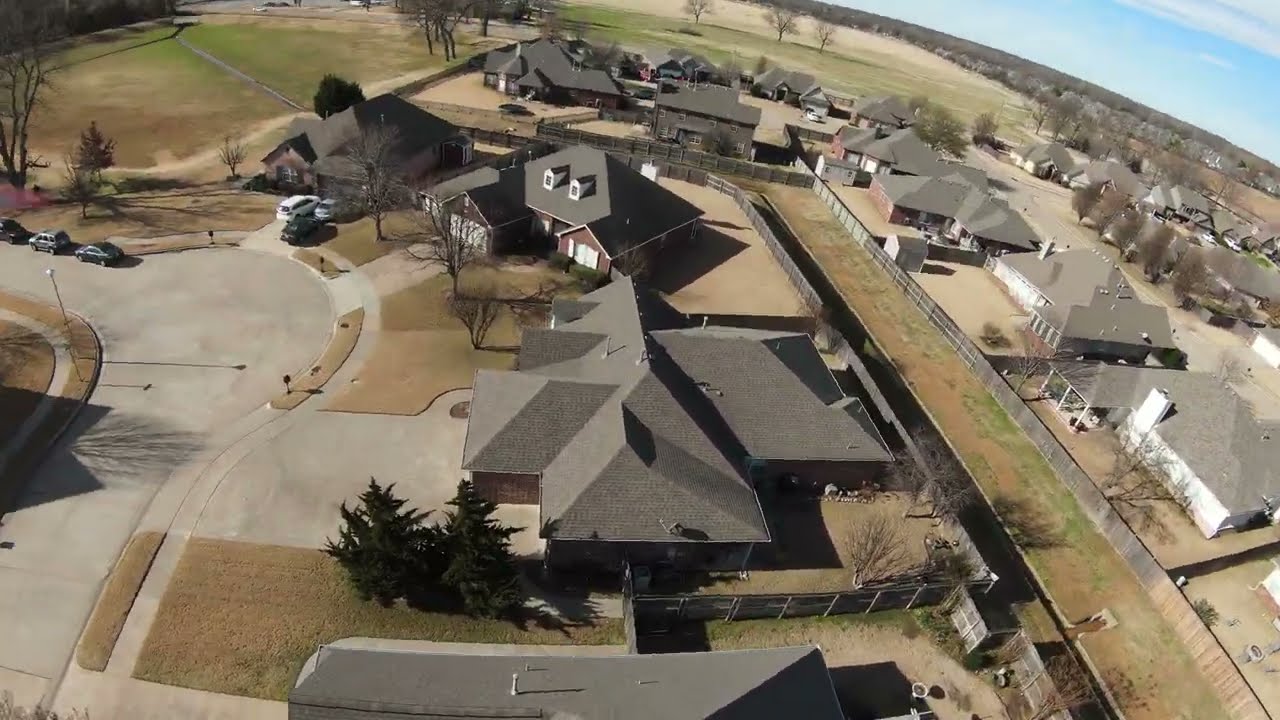This overhead, drone-captured image showcases a newly developed suburban neighborhood filled with large, family-sized homes. The photograph, taken at a slight angle, reveals various homes, most of which share similar architectural features such as single-story layouts with A-frame roofs descending to the garage lines. The majority of these houses have dark gray roofs and brown-colored walls, contrasting slightly with other nearby white houses, but all contributing to a cohesive community aesthetic. Surrounding the homes are well-maintained, yet currently brown lawns, suggestive of fall or winter conditions. The neatly manicured grassy areas and the presence of some pine trees, interspersed with leafless deciduous trees, add a touch of nature to the setting. The houses are separated by small grassy walkways and fenced backyards, with a possible easement for utility or delivery access running along the rear. The neighborhood features nicely paved roads and driveways, further emphasizing its new, well-organized, and uniform development. The absence of a city skyline backs the suburban tranquility, complemented by a clear, unobstructed sky.